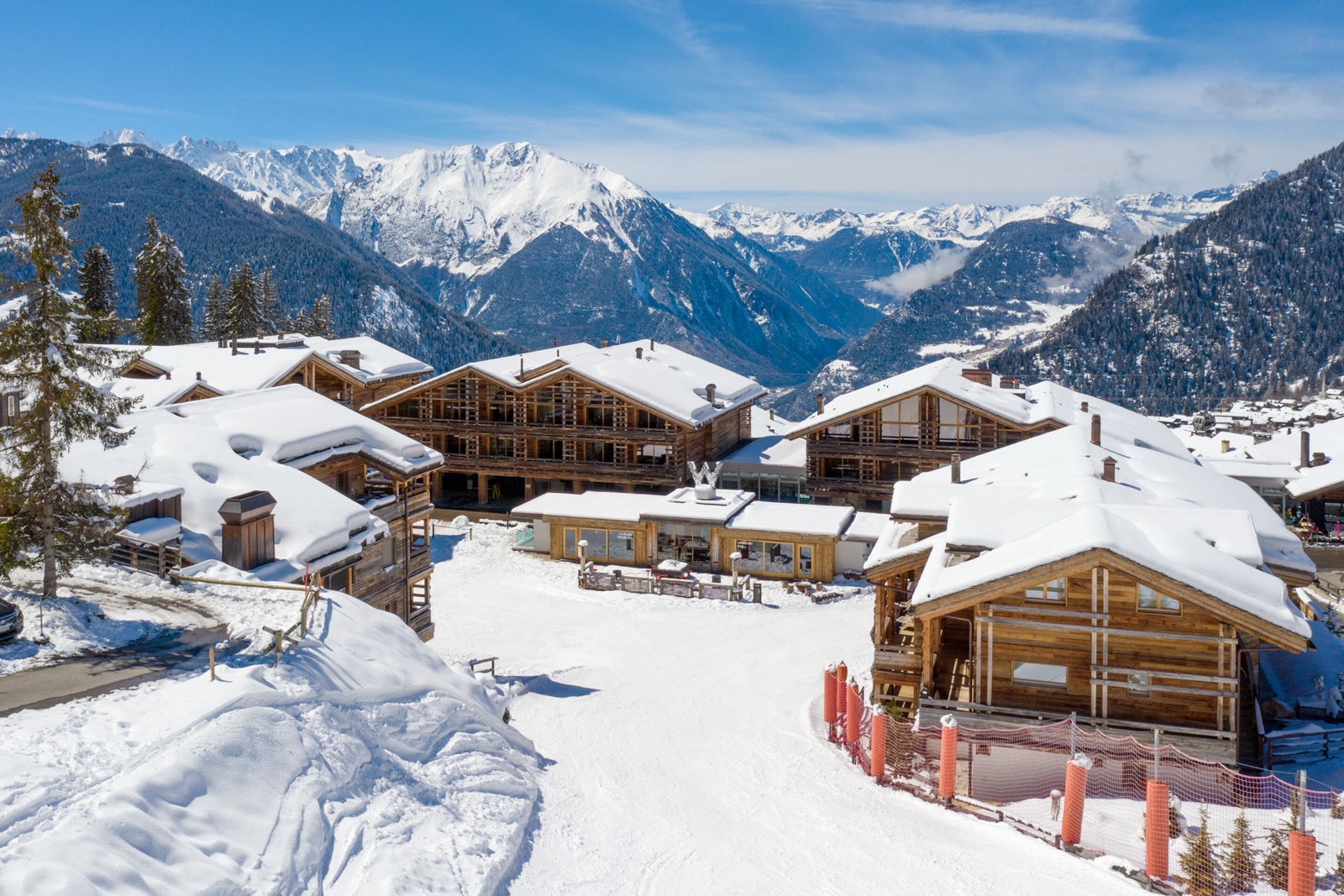This image captures a picturesque ski resort nestled atop a mountain. The backdrop features a stunning dark blue sky adorned with layers of white clouds. The expansive scene includes towering, snow-capped mountains and lush evergreen trees. The foreground reveals a snow-covered road leading to a cluster of wooden buildings, likely ski lodges or hotels, constructed from light brown lumber and featuring pitched roofs laden with snow. Some buildings have chimneys and quaint wooden porches with stairways.

A notable detail is the orange poles with a snow fence on the right side of the image and a snow-packed road on the left. The lodges form a right angle around the mountaintop, suggesting a communal area. Centrally located is a smaller, flat-roofed building that appears to function as a welcome center, marked by a distinct "W" sign indicative of a W Hotel, known for its upscale yet modern appeal. The entire resort area, devoid of visible people, epitomizes a serene winter retreat amidst breathtaking natural beauty.